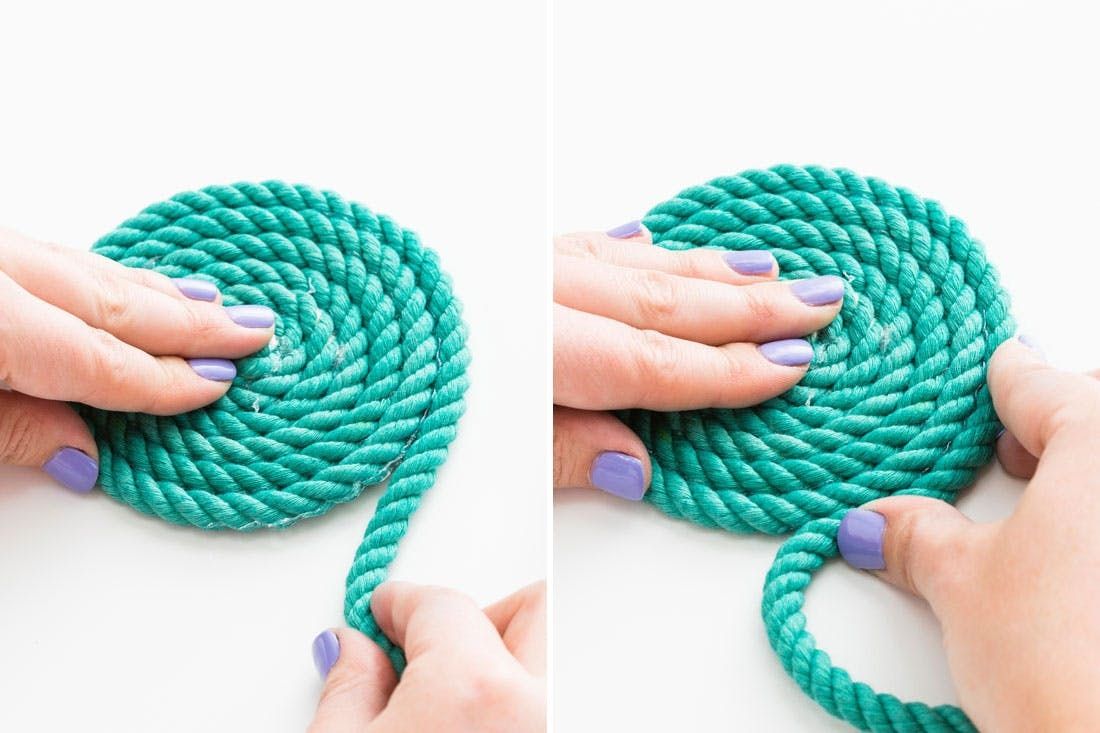The image consists of two side-by-side photographs separated by a white line, each featuring a Caucasian woman’s hands working on coiling a thick, turquoise rope against a white background. In the left photograph, the woman’s left hand holds the middle of the rope down with three fingers, while her thumb is positioned on the edge and her right hand holds the free end of the rope. Her fingernails are short, manicured, and painted with a purple polish. The rope is wound tightly into a large circle, partway through the coiling process. In the right photograph, the woman’s left hand maintains pressure on the newly tightened, thicker coils, this time using her pinky on one edge and three fingers in the center, while her thumb still grips the outer edge. Her right hand is securing the outermost layer of the coil. The rope arrangement gives the impression of a detailed instructional process, showcasing the progression and meticulous technique involved in creating the coiled rope mat.